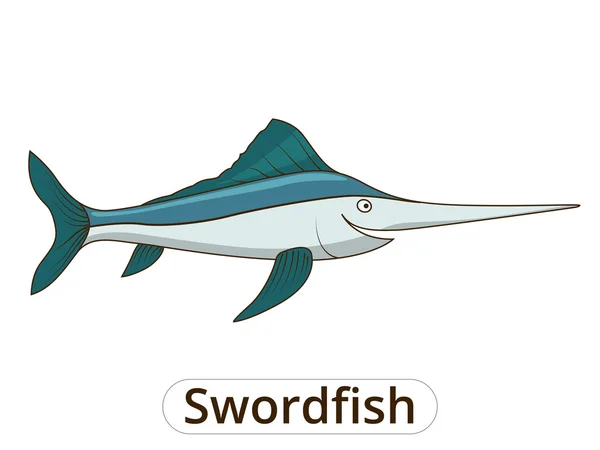The image depicts a cartoon illustration of a swordfish against a solid white background, facing the right side with its long, pointed nose extending prominently. The fish features a small circular eye with a dot, situated above its mouth, which is open in a manner that almost resembles a smile. The body of the swordfish is detailed with multiple colors: the top part is a mix of bluish, tealish hues, including two shades of blue for added depth, while the belly and nose are rendered in two shades of gray. The dorsal fin, tail fin, and other swimming fins are shaded in a greenish blue or teal color. These fins include a long, prominent fin running along the back and smaller fins near the neck and tail area, with the tail fin distinctively split in two. Below the fish, the word "swordfish" is displayed in large black letters within a tag-like shape that has a thin black outline and a light gray border. The "S" in "swordfish" is capitalized, emphasizing the name.